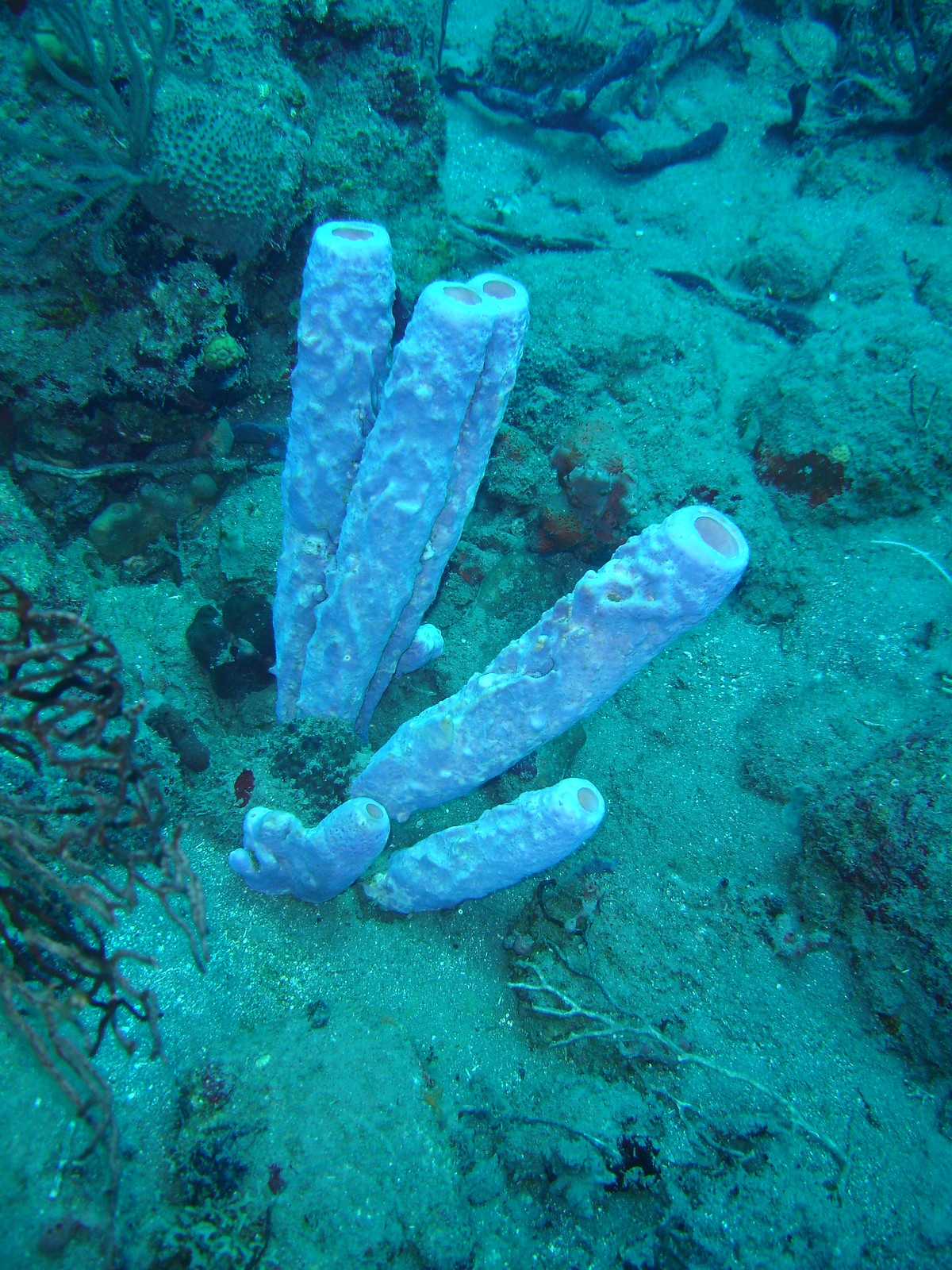This photo captures an underwater scene taken several feet beneath the surface, where sunlight trickles down to illuminate the seabed. The predominant color tone of the image is aquamarine blue, creating a subdued, monochromatic effect. The focus is on several tubular, cylindrical objects that resemble segments of a coral reef. These formations are a light blue, almost baby blue, with a rough texture akin to dried, paint-dipped rollers. There are six main tubes: four are tall, with three clumped together at the center and the fourth leaning away. The remaining two tubes are shorter, positioned beside the leaning one.

The seabed beneath these formations is sandy, interspersed with rocks, little sea formations, and patches of algae. Further back, various plants cling to the reef, including veiny, sponge-like structures, enhancing the dense, yet serene underwater environment. Although the overall picture lacks vibrant colors, the contrast between the rich blue cylindrical coral and the surrounding greenish-blue water adds a subtle depth to the photograph.